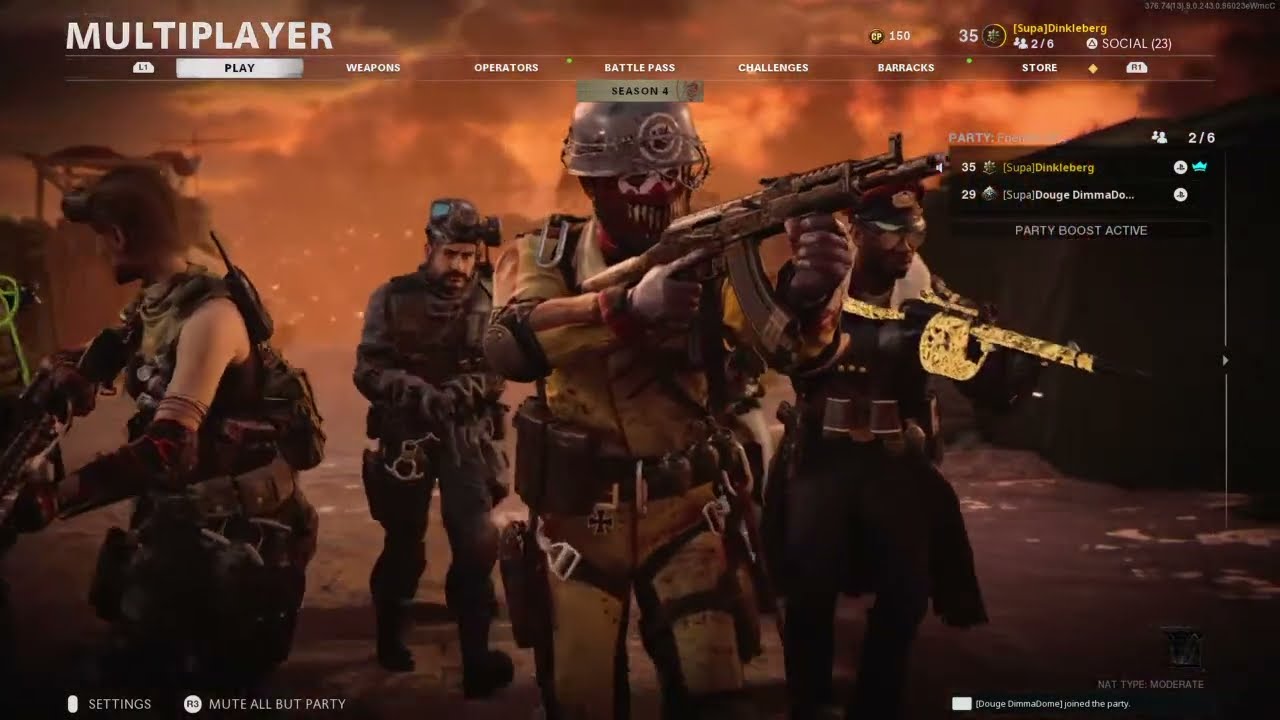In this detailed screenshot from an online multiplayer warfare video game, four characters stand poised for battle on a debris-littered pavement, framed by an apocalyptic orange sky filled with smoke and a burning backdrop. Dominating the foreground, the main character is clad in a tan full-length bodysuit with a gray helmet, a striking red face mask adorned with white teeth and eye outlines, and a black utility belt. He grips a gun holstered at his shoulders. Flanking him are diverse characters: to the far left, a woman in a sleeveless shirt and forearm warmers glances back over her right shoulder, exuding readiness. Behind the central figure, on the right, an African-American male sports a red cap, sunglasses, a long overcoat, and wields a vintage Gatling gun. To the left, another male character in gray utilities with a gas mask on his head, his pale skin accentuated by a long mustache, completes the quartet. The game's interface is visible in the upper left corner, prominently displaying the word "multiplayer" along with tabs for play, weapons, operators, battle pass, challenges, barracks, and store. The setting, evocative of a war zone, suggests these characters have just disembarked, ready to engage in combat.